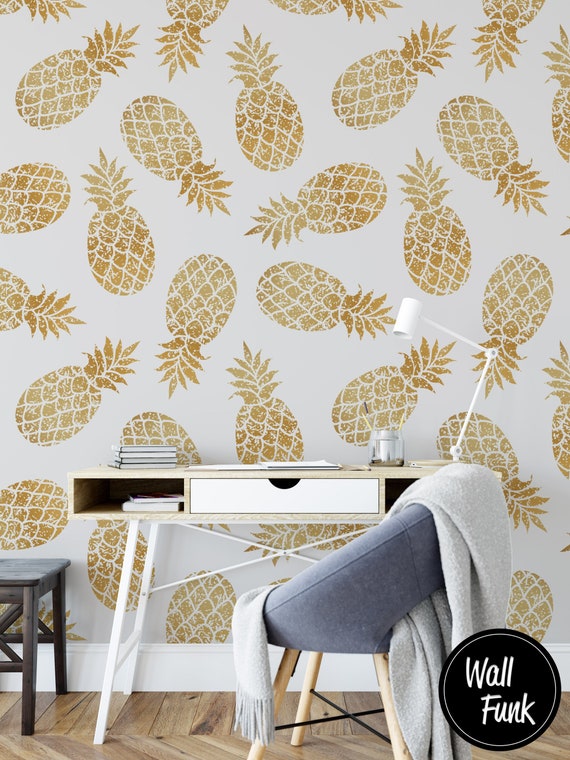The image depicts a cozy setup featuring a small, light-colored, rectangular desk positioned against a wall adorned with white wallpaper covered in numerous gold pineapple patterns, each with intricate white line details for texture. The desk includes a white pullout drawer with two small cutouts on each side, with at least one book visible inside. Resting on the desk is a sleek, white L-shaped arm desk lamp, not currently illuminated, and a stack of books on the left side. Accompanying the desk is a cushioned, donut-shaped gray seat with four wooden peg legs, draped with a cozy white afghan blanket. To the left and partially visible, a dark wooden stool sits on a zigzag patterned wood tile floor. Adding a modern touch, a bold black circle in the lower right corner of the image displays the brand name "Wall Funk" in white letters.